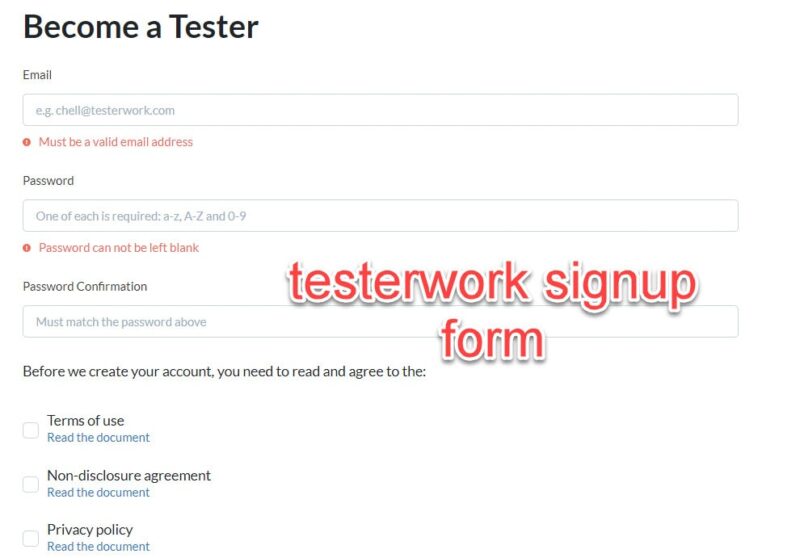The webpage displayed is a sign-up form for individuals interested in becoming testers. At the top of the page, there is a prominent heading in black, bold text that reads "Become a Tester." Below this heading, users are prompted to enter their email addresses. There is a text field with a placeholder example email, "chelll.testerwork.com," and beneath it, a red warning message indicating that the email address must be valid.

Further down, the page includes a password field with instructions stating that the password must contain at least one lowercase letter (a-z), one uppercase letter (A-Z), and one number (0-9). A red warning message alerts users that the password cannot be left blank. Adjacent to this is a password confirmation field, with a note in red text indicating that the password must match the one entered above.

Before account creation, users are required to read and agree to several documents. There are three sections, each accompanied by a checkbox: "Terms of Use," "Non-Disclosure Agreement," and "Privacy Policy." Each section has a corresponding link in blue text labeled "read the document."

To the right of the page, there is a visually distinct, large red button with white text that reads "Test Your Work Signup Form," signaling users to proceed with the sign-up process.